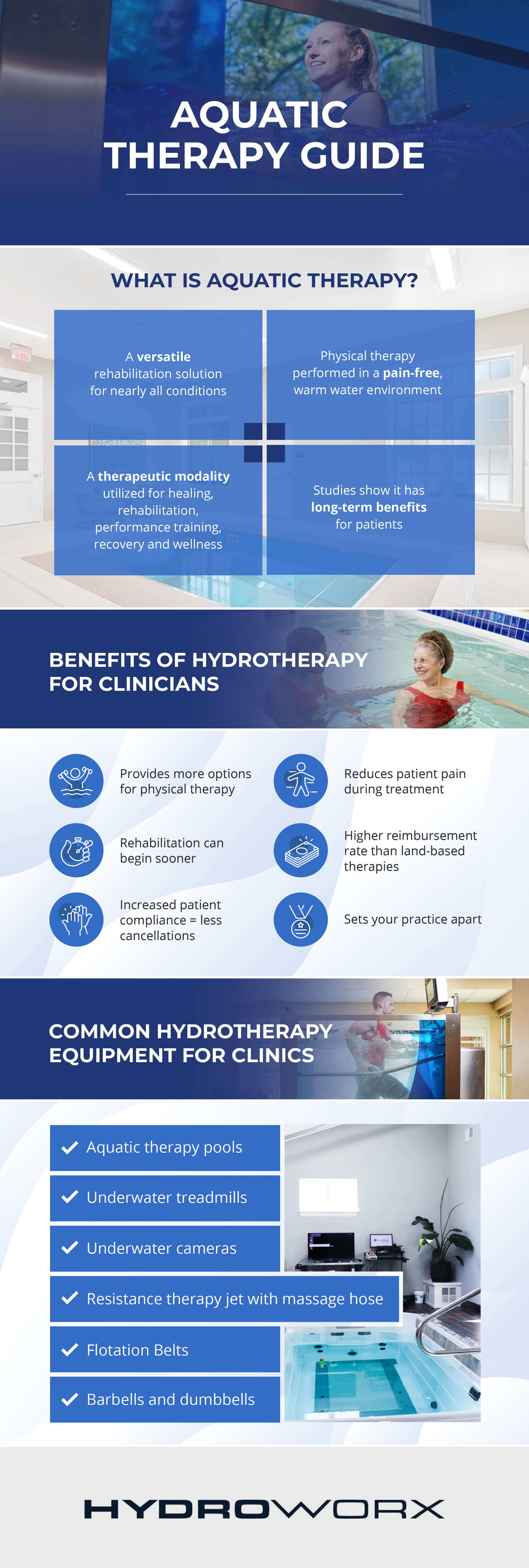This infographic, created by HydroWorks, serves as a detailed Aquatic Therapy Guide, all set against a clean white background with a cohesive color scheme featuring shades of blue and white. The top section prominently displays an image of a woman, beneath which the bold title "Aquatic Therapy Guide" is printed. 

The guide begins by explaining "What is Aquatic Therapy," emphasizing its versatility as a rehabilitation solution and its implementation as physical therapy in a warm, pain-free water environment. This section highlights its use for healing, rehabilitation, performance training, recovery, and overall wellness, noting that studies have shown long-term benefits for patients.

Further down, the infographic outlines the "Benefits of Hydrotherapy for Clinicians," accompanied by an image of people happily engaging in aquatic therapy. It lists advantages such as providing more options for physical therapy, allowing for earlier rehabilitation, reducing patient pain during treatment, increasing patient compliance thereby reducing cancellations, and setting the practice apart from competitors.

The final segment, labeled "Common Hydrotherapy Equipment for Clinics," is introduced with an image of a person undergoing rehabilitation in water. It enumerates essential equipment, including therapy pools, underwater treadmills, underwater cameras, resistance therapy jets with massage hoses, flotation belts, barbells, and dumbbells.

Throughout, the infographic features images and detailed descriptions to aid in visual understanding, making it a comprehensive resource on aquatic therapy.